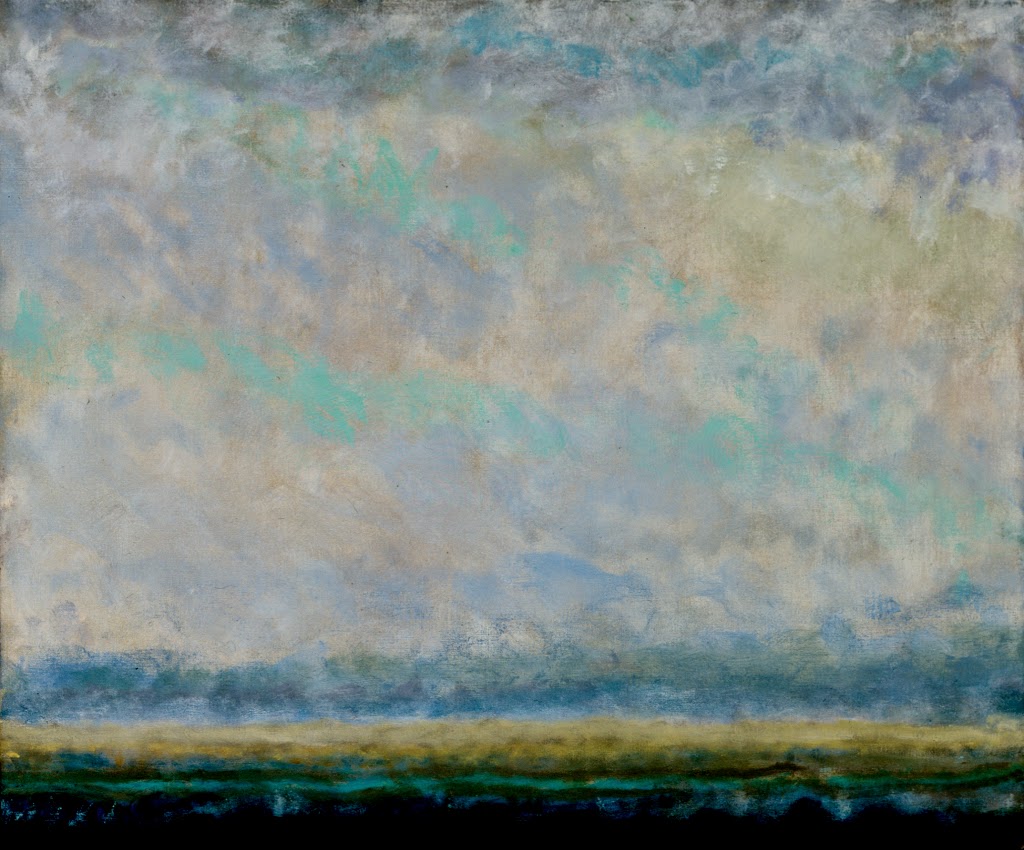This painting, reminiscent of an impressionistic style akin to Monet, depicts an abstract outdoor scene primarily dominated by a sprawling, intricate sky. The focus is on the sky, forming about three-fourths of the composition, showcasing a dramatic play of colors and cloud formations. At the top, a dark blue expanse gives way to layers of white clouds separated by bands of lighter blue and teal tones. Interspersed throughout are splotchy areas of gray and darker blue, adding depth and movement. Below the sky, a blurry green area suggests the presence of grass or trees, grounding the scene. The very bottom of the painting features a series of horizontal bands: a brown strip that might represent soil, a thin light blue line possibly indicating a stream, and an even darker brown band at the base, adding to the abstract nature of the landscape.